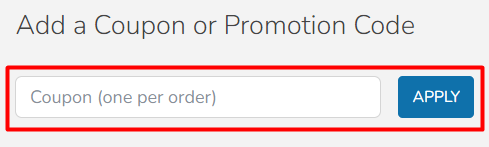This image shows a cropped section of a website's checkout page, indicative of an online store. The background of the image is a light smoke gray color, giving it a neutral tone. The overall shape of the image is rectangular.

At the top of the image, there is a black text instruction that reads "Add a coupon or promotion code." Beneath this text, a red box highlights the area designated for entering the coupon code. This red box surrounds both the input field and the button used to apply the code.

The input field itself has a white background and contains the placeholder text "Coupon one per order." Adjacent to this field on the right side, there is a blue button with white text that says "Apply."